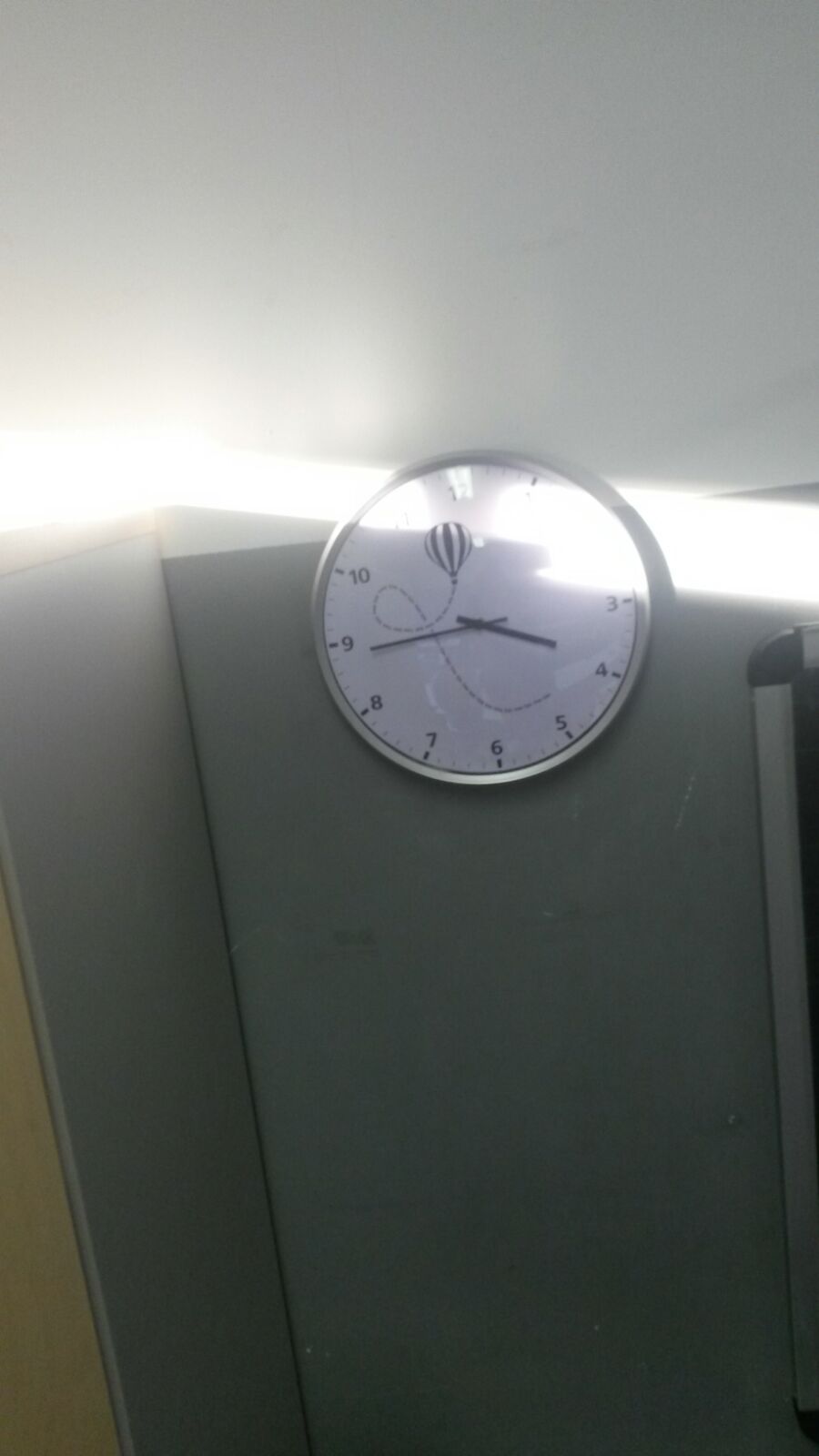In an office cubicle with a dark grey wall and a band of light dividing it from the white ceiling, a silver-framed circular clock hangs prominently. The clock's face is white with black hands and numbers, displaying the time as approximately 3:45. A streak of sunshine illuminates the area around 11, 12, and 1 on the clock. Additionally, a black and white hot air balloon is depicted near the number 12, with a dotted line swooping down and looping around to connect to the number 4.